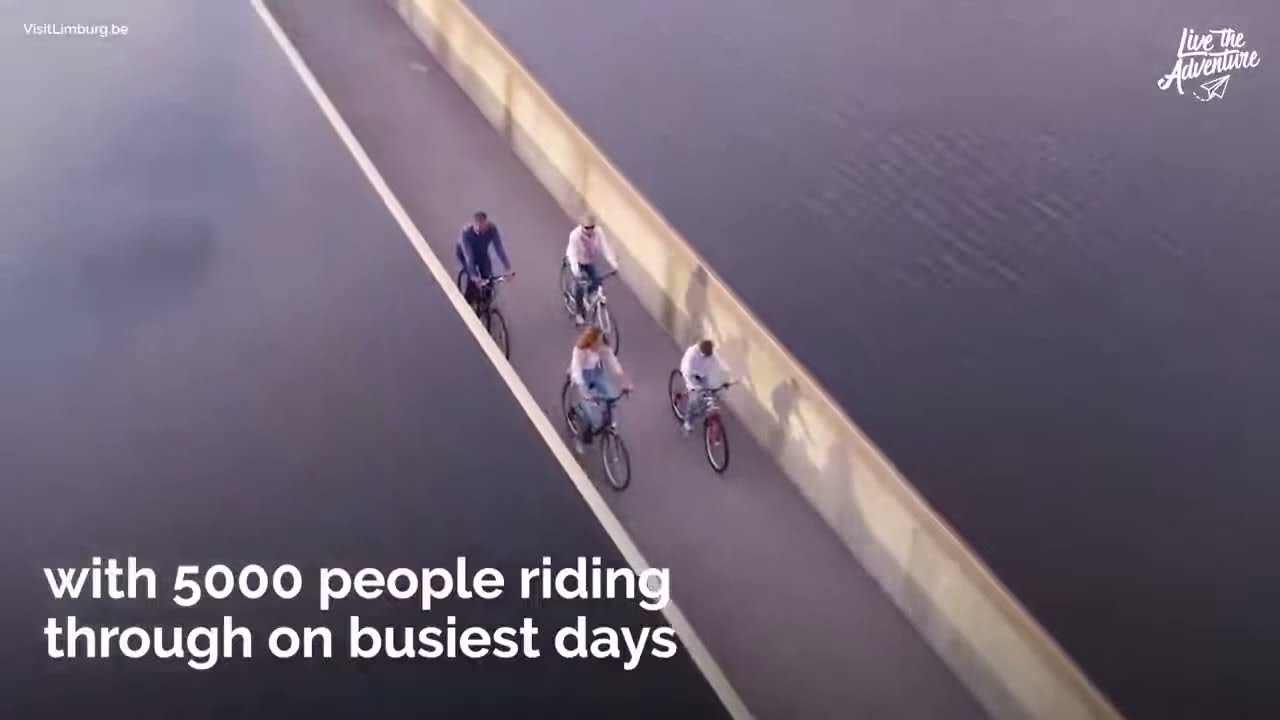The image is a detailed advertisement for VisitLindbergh.be, promoting a scenic bikeway popular for both tourism and exercise. In the foreground, four people riding bicycles can be seen; the bikeway is elevated above a body of water, noticeable by the ripples on the right. The bikeway itself is gray, narrow, and not suitable for cars. The cyclists include a young girl in the front, her younger brother, and two adults behind them, one wearing a white top, and the other a purple shirt. In the lower left corner, white text states, "With 5,000 people riding through on the busiest days." The upper right corner features cursive text, "Live the Adventure," accompanied by a graphic of a paper airplane, accentuating themes of movement and enjoyment. The upper left corner has the website "visitlindberg.be" in small white letters, indicating an international destination. The palette of the image consists primarily of gray, light yellow, and white tones, adding to its inviting and adventurous allure.